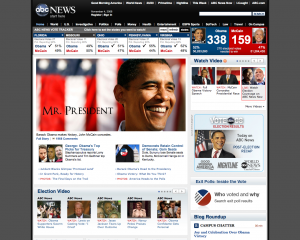A detailed screenshot from the ABC News website during Barack Obama’s presidential campaign is depicted. The central part of the image shows the actual ABC News webpage, surrounded by a gray background on both sides, indicating that the webpage has been significantly reduced in size, rendering much of the text illegible. At the top of the webpage, there are electoral polls visually represented, with a series of five total poll boxes displaying red and blue colors, likely symbolizing Republican and Democratic candidates. Notably, four of the blue-colored boxes have check marks next to them, indicating a lead for the Democrats.

Below this, there is a prominent poll showing a head-to-head comparison, featuring a clear image of Barack Obama, labeled with the number 338, and another male candidate in a red box labeled with the number 159, presumably indicating the electoral votes. Beneath this poll is a notable image of Barack Obama, standing confidently against a backdrop of the American flag with the title "Mr. President" beside him. Obama is depicted smiling and looking off to the right.

Further down the page are two news article thumbnails, although they are too small to decipher the exact content. At the very bottom of the screenshot, there appears to be a series of election-related video thumbnails, hinting at comprehensive coverage of the presidential election.